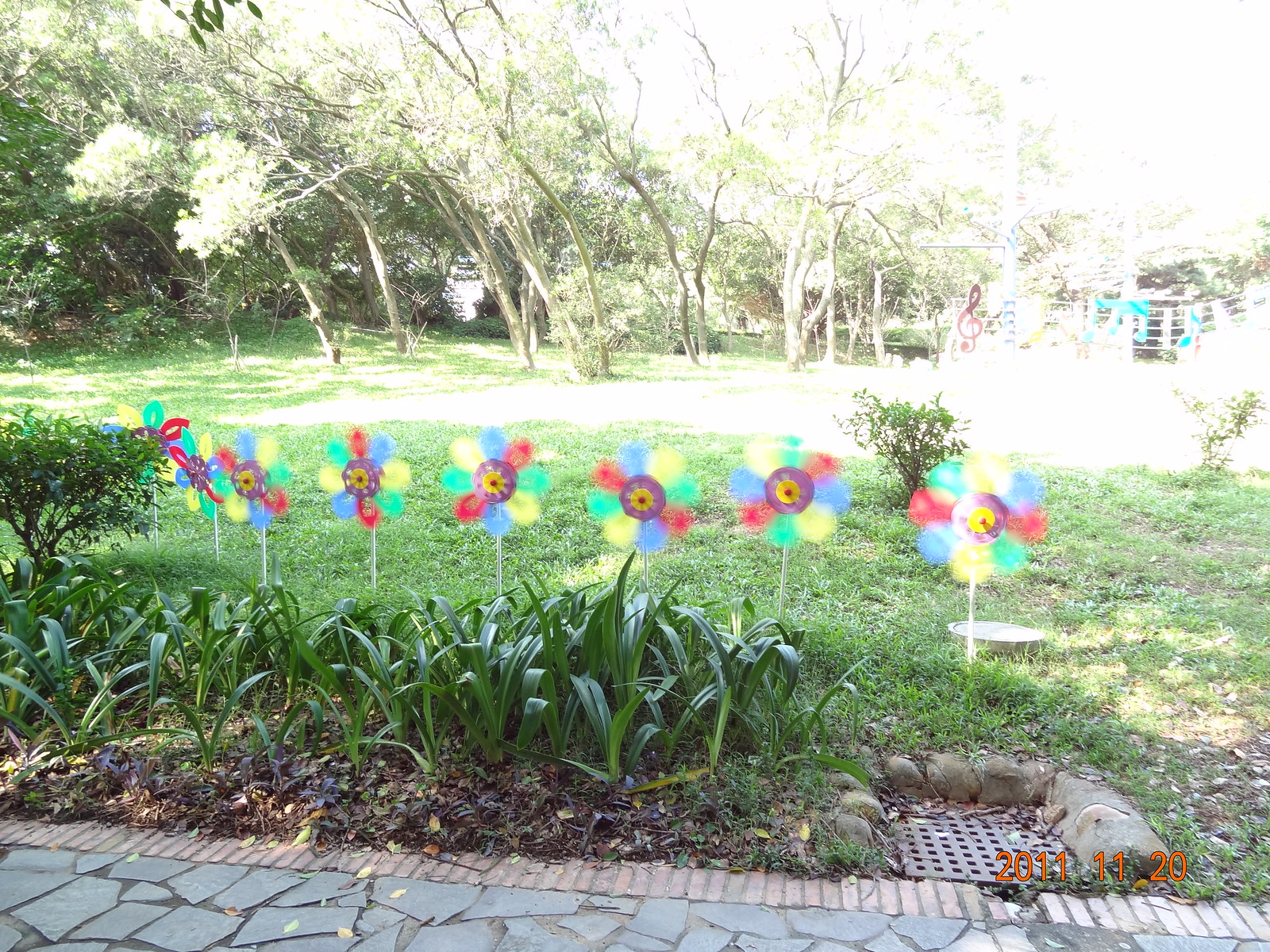The image captures a lively backyard garden scene. In the foreground, a slightly diagonal stone walkway lines up with bricks, leading the eye through the garden. At the bottom right, an orange date stamp reads "2011-11-20" next to a drainage area. Surrounding the path are lush, leafy green plants among which a row of colorful pinwheels—adorned in white, red, green, blue, purple, gold, and yellow—spin in the wind. Further back, a flower bed showcases a variety of vibrant plants nestled in mulch. To the right, musical notes and a treble clef, presumably part of decorative banners or art pieces, add a whimsical touch, though partially washed out by the bright sunlight. The background features a sprawling yard filled with green grass and arching trees, framing the idyllic setting.